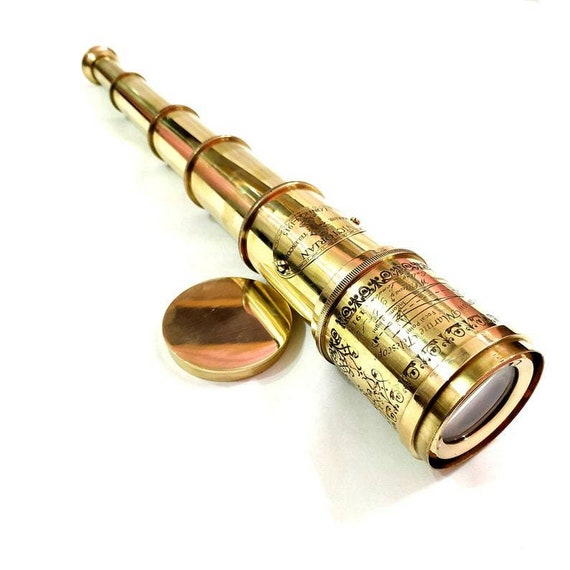This image showcases an antique, ornate golden telescope resting against a transparent background. The telescope, likely similar to those used by pirates, features intricate black engravings and writings that extend around its top portion, including a blackened oval plaque attached with screws. The telescope is fully extended, revealing its six segmented, retractable parts, culminating in an eyepiece at one end and a white inner lens at the other. Positioned at a 45-degree angle, the larger part of the telescope stretches to the lower right-hand corner of the frame, while the eyepiece points towards the upper left. Sitting adjacent to the telescope is its cap, slightly to the side, adding to the overall vintage and sophisticated appearance of the device. The entire image is set against a stark white backdrop, enhancing the detailed craftsmanship of the telescope.